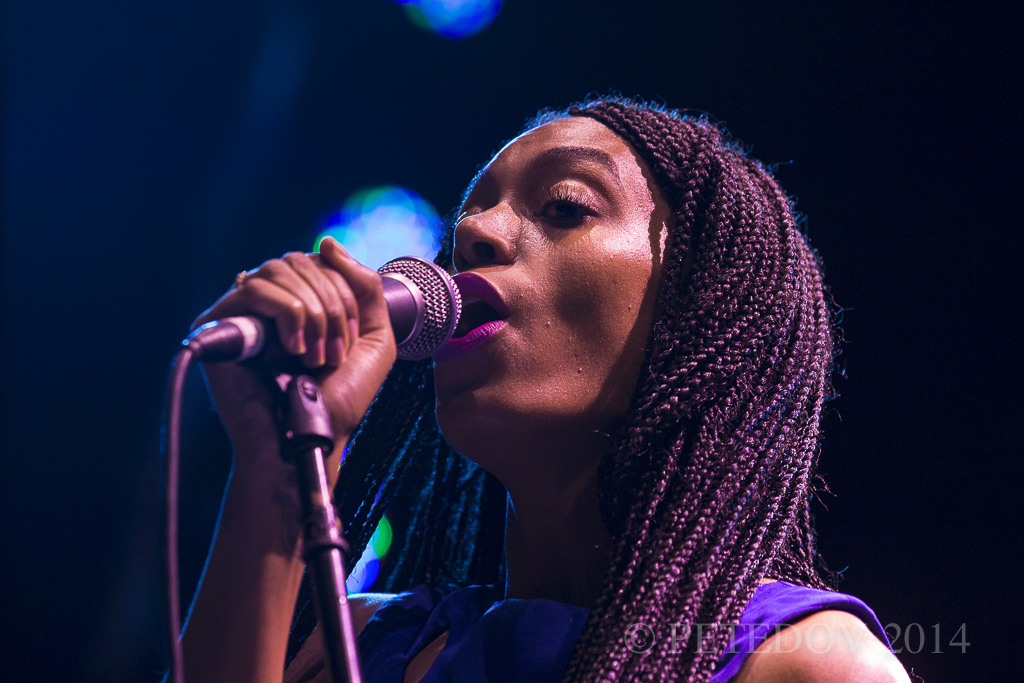The image depicts a black woman with intricately braided hair, appearing to have a purple hue, standing on a stage against a dark background. She wears a sleeveless, bluish-purple dress and pink lipstick. With her right hand, she grasps a stand microphone, poised near her open mouth, suggesting she is singing. She gazes slightly to her left. Several blurred blue lights illuminate the background, creating a striking contrast. The photo captures her from the top of her head to her chest. In the bottom right corner, the photo is marked with copyright information, reading "PETEDON 2014" or "FEDER 2014."